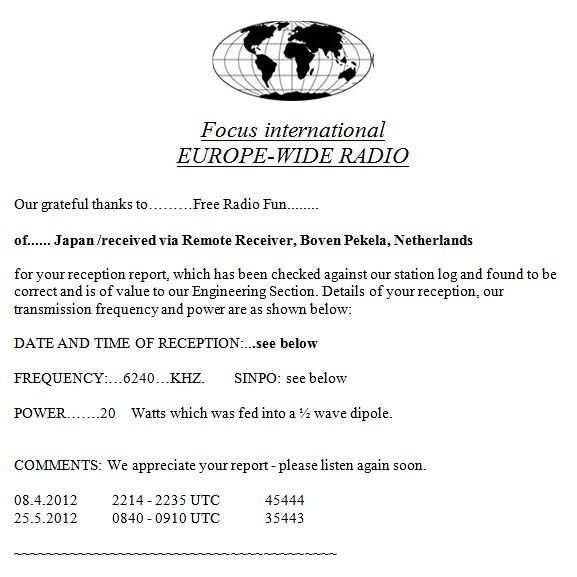The image depicts a detailed black and white letter set against a solid white background. At the top of the letter, there is an oval globe illustration highlighting various countries in black with visible longitude and latitude lines. Beneath the globe, in gray lettering, it reads "Focus International" followed by "Europe-wide Radio" in larger, underlined black text. The main body of the letter expresses gratitude to "Free Radio Fun of Japan," acknowledging the reception report received via a remote receiver in Boven-Pakala, Netherlands. The report has been verified against the station log, confirmed as correct, and noted to be valuable to the engineering section. Detailed information about the reception, including the date, time, transmission frequency of 6240 kHz, and power output of 20 watts, is listed below. Additionally, there are comments expressing appreciation for the report and an invitation to listen again soon, followed by specific reception dates and times: April 8, 2012, at 2214-2235 UTC with reception quality marked as 45444, and May 25, 2012, at 0840-0910 UTC with reception quality marked as 35443. The letter has the appearance of a postcard likely mailed out by the radio station.